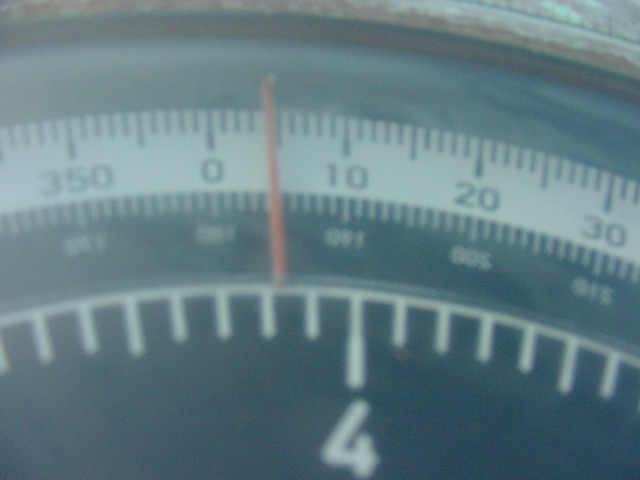This horizontal photograph captures an extremely close-up and blurry image of a rounded gauge. At the bottom of the gauge, the number "4" is prominently displayed, surrounded by incremental gauge lines where a pointer would typically be positioned. Above this, a smaller section features increasingly dense and detailed lines, including a noticeable red gauge line. Just above this area, a black section with very fine lines is visible, although the numbers are unreadable due to the blurriness.

Moving higher, the lines become more spaced out and discernible. On one side, the number "350" is visible, along with incremental markings of "0," "10," "20," and "30." The entire gauge seems to potentially go up to "400" units. The gauge is set within a metal casing, enhancing its rounded appearance. Notably, the segment displaying the large "4" does not reveal any additional numbers or indications clarifying the gauge's specific purpose, whether it measures temperature, speed, or another parameter.